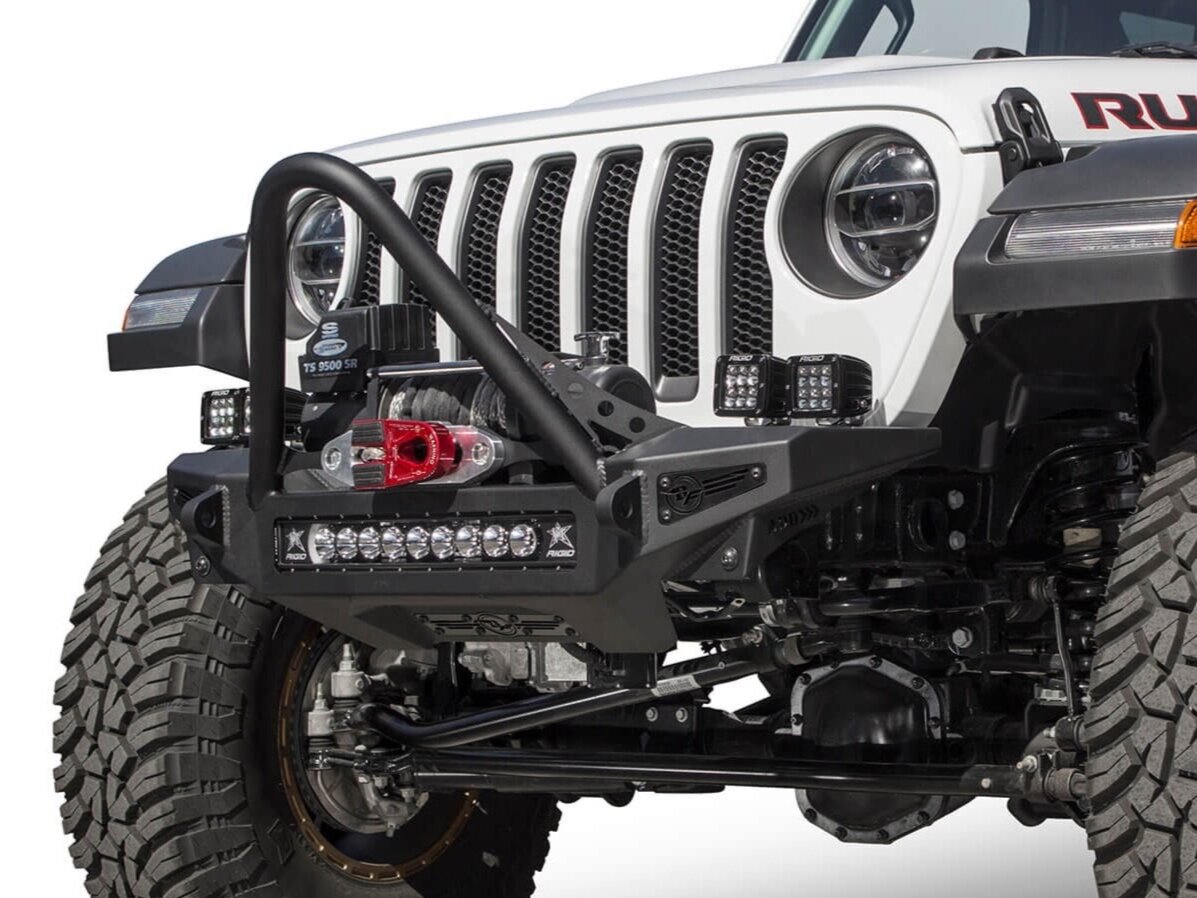This color photograph presents a close-up view of the front end of a white Jeep, possibly a Wrangler or a newer model, showcasing its rugged features and advanced modifications. Prominently displayed on the side of the hood are the letters "RU" in black with a red outline, likely indicating the Rubicon model. The Jeep's front hitch is equipped with a robust electronic winch, featuring a thick rope that is spooled and ready for heavy-duty use. Adjacent to the winch is a mysterious red device, possibly a guide or fairlead for the rope. Below the winch is a row of LED lights, emblazoned with a star image and some indiscernible white text, providing additional illumination. Crowning the front are two larger, box-shaped light assemblies, each housing twelve individual lights arranged in four rows of three, enhancing visibility. The vehicle is fitted with oversized, black all-terrain tires with deep treads, hinting at its off-road capabilities. The visible enhancements include an improved suspension system with prominent shocks and spring coils, allowing a glimpse at the meticulous engineering beneath the Jeep's tough exterior. The image captures only up to the lower part of the passenger window and just above the dashboard, focusing attention on the rugged front grill, headlights, and intricate details of the Jeep’s formidable front end.